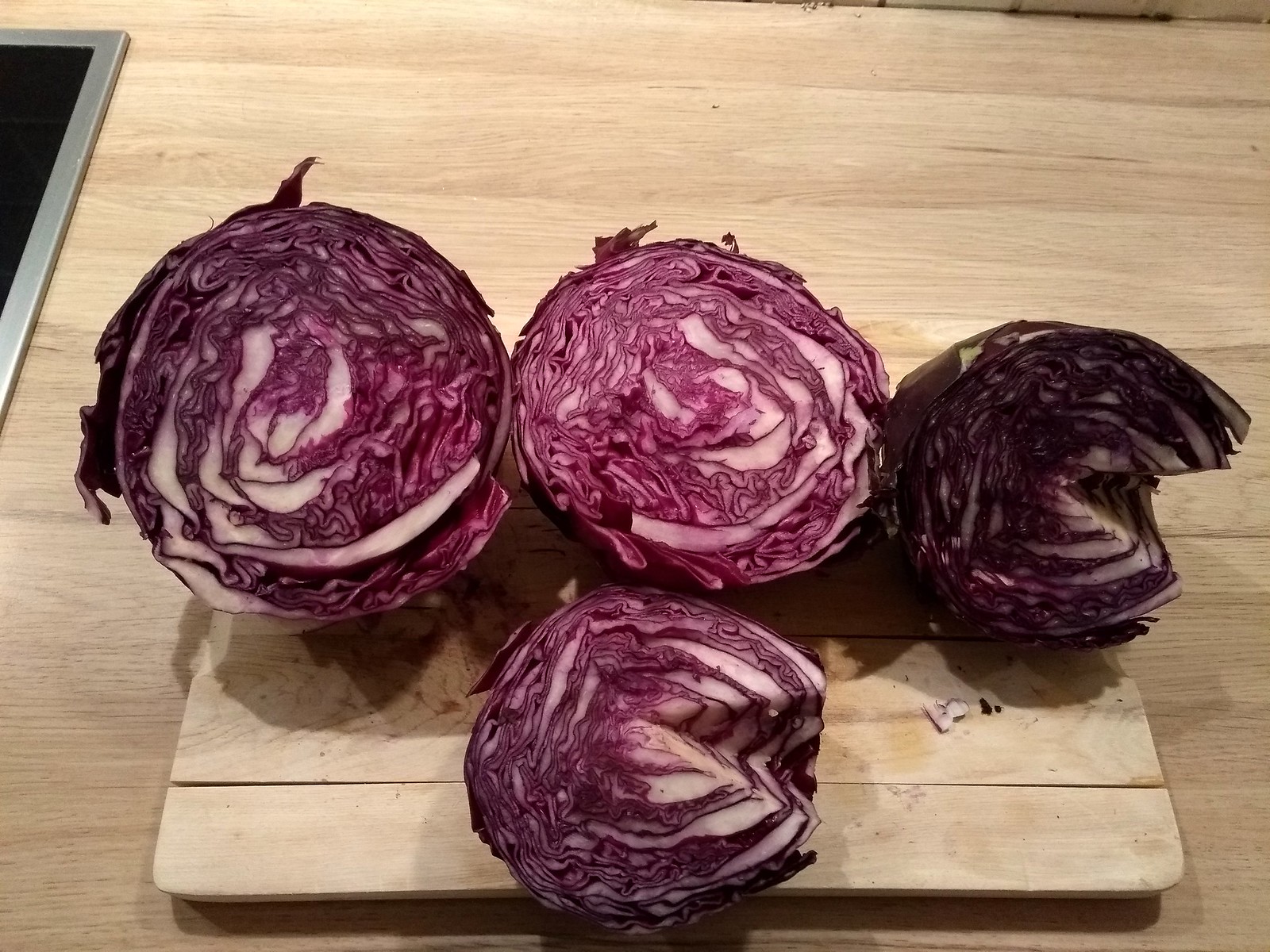This photo showcases four vibrant heads of red cabbage, each sliced in half, arranged on a rustic wooden cutting board positioned atop a butcher block countertop. The cutting board itself appears slightly weathered, with a seam visibly separating. The cabbages vary slightly in size and shade, exhibiting a spectrum of deep reds and purples interlaced with crisp, white veins. Dominating the left side is a large head of cabbage, followed by another sizable one in the middle, and a notably darker, almost maroon head on the right. A smaller head sits in the foreground. Both the foremost and the rightmost heads display distinctive V-shaped cuts where their stalks were removed. The scene is framed by the subtle detail of chrome trim along the edge of the countertop, adding a hint of modernity to the otherwise earthy setting.